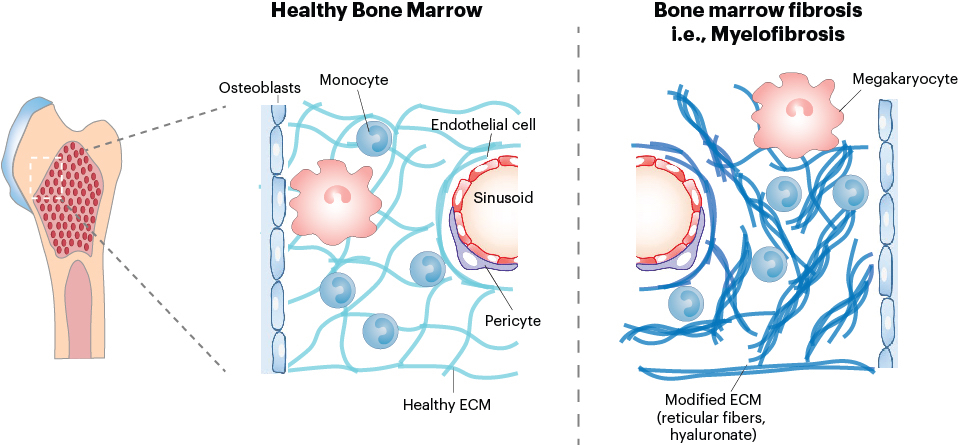This image, set against a white background, appears to be an illustration from a medical textbook, depicting two states of bone marrow within a femur cutaway. The left side illustrates healthy bone marrow, labeled at the top, featuring the upper part of a femur in a beige tone. Inside, it showcases a cross-section filled with clusters of red circles pointed out as osteoblasts. Additionally, there are labels identifying other components like monocyte, endothelial cell, sinusoid, pericyte, megakaryocyte, and healthy extracellular matrix (ECM). Blue squiggly lines and pink dots illustrate these elements in a simplified and color-coded format. The right side presents a similar illustration but highlights bone marrow fibrosis (myelofibrosis), as indicated at the top. This part features more dense and numerous blue squiggly lines, representing reticular fibers and modified ECM, which clearly contrast with the healthy section by demonstrating the pathological changes characteristic of myelofibrosis. The detailed differences emphasize the impact of fibrosis on bone marrow structure and function.